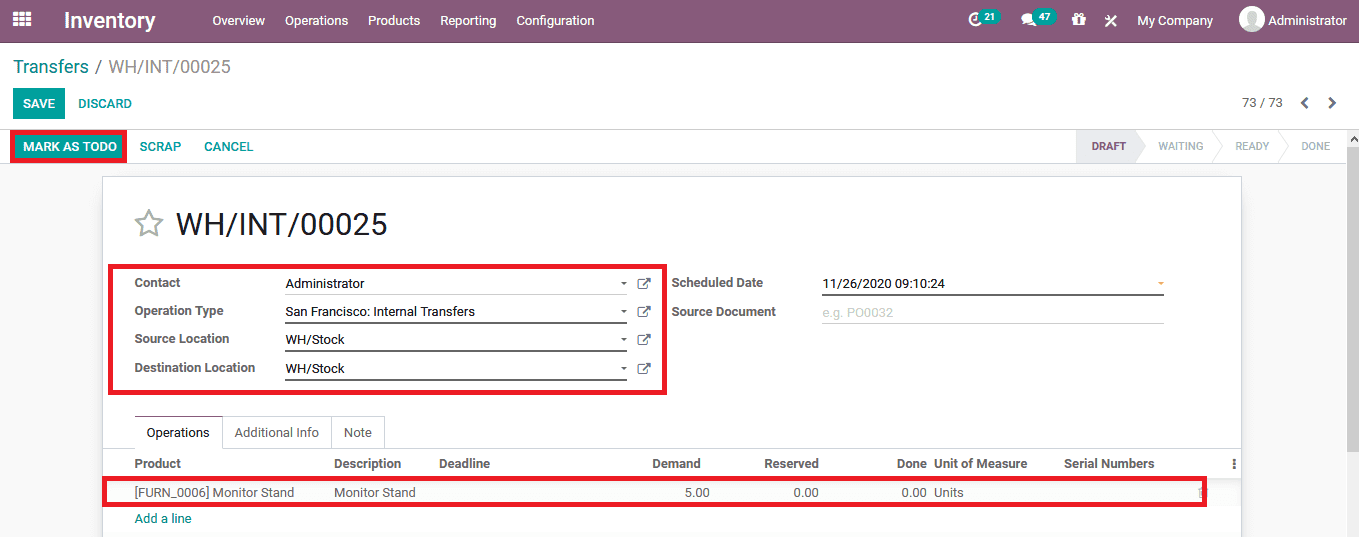The website interface displays a prominent purple navigation bar at the top, with white text for menu options listed side by side. On the left, there is a square divided into six smaller boxes. To its right, a section titled "Inventory" can be seen. The navigation bar includes options labeled "Overview," "Operations," "Products," "Reporting," "Configuration," and on the far right, there's an icon with a blue circle indicating 24 message notifications and another circling number in the 40s, followed by an 'X'. Adjacent to these, a 'My Company' section is visible alongside a white circle labeled "Administrators."

Beneath the purple navigation bar, there is a blue sub-bar featuring options such as "Transfers," "Save," "Discard," "Mark As To Do," "Scrap," and "Cancel." This section also includes categories like "Drafts" and "Waiting."

Below this, another prominent square displays the identifier "WH/INT/00025." Directly below this, a detailed list with a red outline includes specific details such as "Contact," "Administrator," "Operation Type," "San Francisco Internal Transfers," "Source Location: WH/Stock," and "Destination Location: WH/Stock."